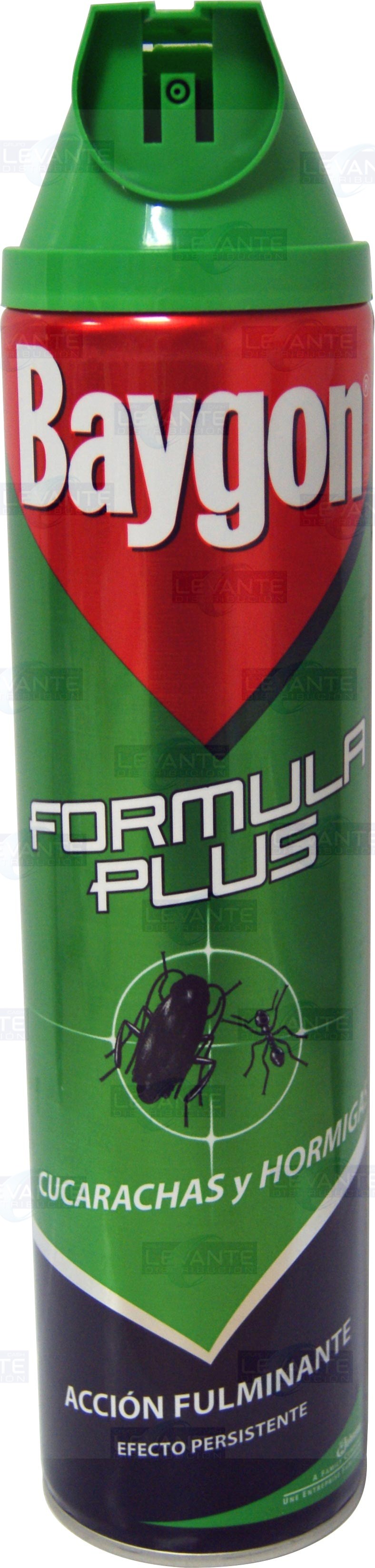This image is a high-quality digital photograph of a product, likely intended for an e-commerce website. The background is pristine white, ensuring that the product stands out prominently. The product is a green can of bug spray, distinguished by its sleek, elongated design. At the top of the can, there is a uniquely shaped triangular nozzle, designed for precision in spraying. The spray opening, which is circular with a central dot, is clearly visible.

The can is an appealing shade of green and features a red, downward-pointing triangle that houses the brand name "Baygon" in large white font. Directly below this, "Formula Plus" is written in white text against the green background of the can. The lower section of the can showcases a black cockroach and a brown ant on the left and right, respectively, with a white trigger hair icon positioned above them, indicating the spray's target pests.

Below this icon, there's text in Spanish written in white font, followed by a small white ribbon leading into a blue section which also contains more Spanish text. Towards the bottom of the can, there is a green banner with additional white text that is difficult to decipher, possibly due to size or resolution limitations. The can also features a logo which appears to end with the letters "NTE," though the full text of the logo is not entirely clear. This can of bug spray is clearly marked, with detailed visuals and text to inform potential buyers of its use and efficacy.